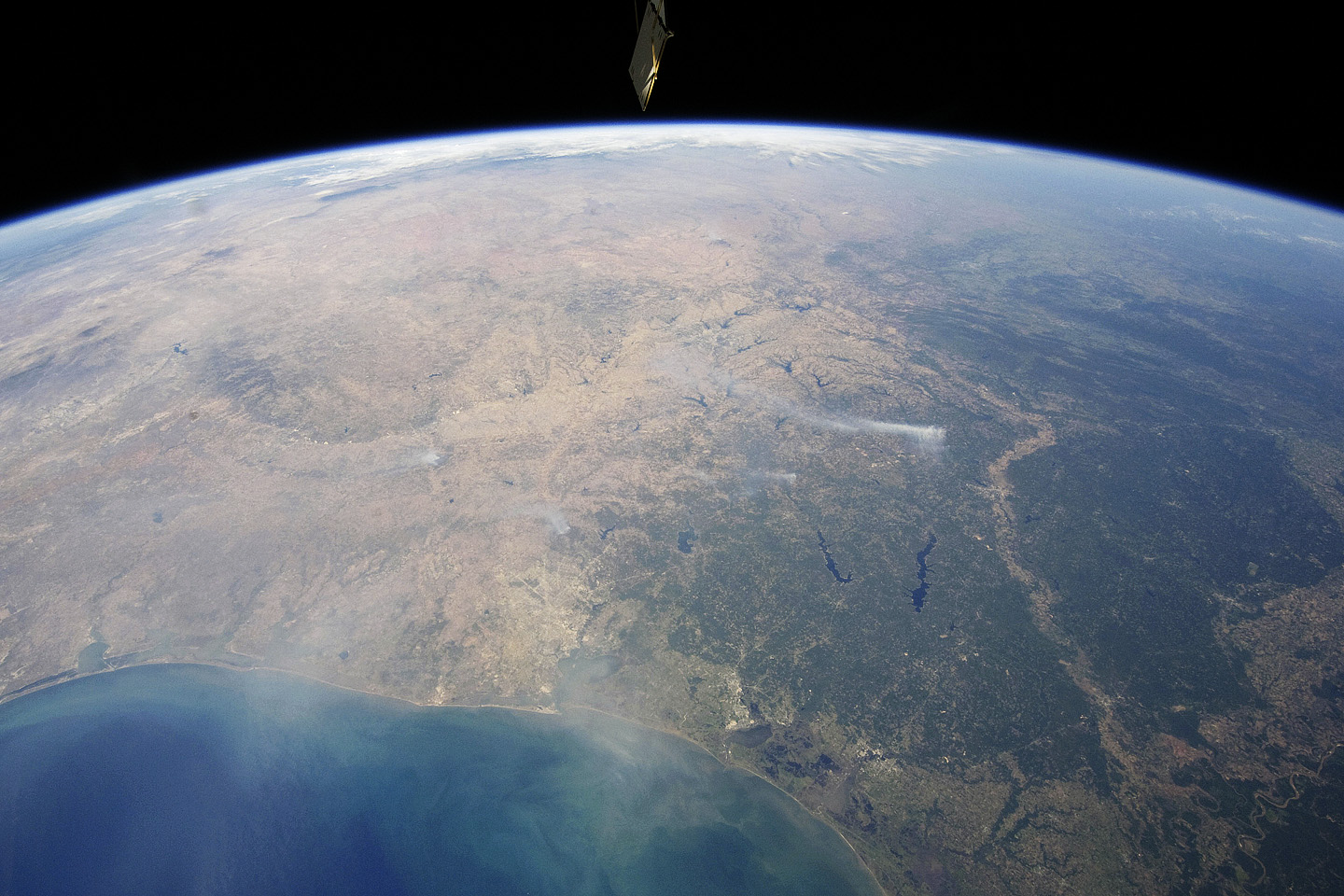This horizontal photographic image, likely taken from a satellite or space station, captures a partial view of Earth. The planet's curvature is evident, with the image being cropped on the left, right, and bottom, creating a curved outline across the top. The Earth's surface displays a mix of blue and brown colors, indicating water bodies and land masses. On the right side, a large expanse of blue suggests an ocean, while the left side features a significant, mostly brown land mass that stretches over roughly two-thirds of the visible area, indicating a desert or dry region. Patches of green are also visible, marking areas of dense vegetation or forests. The background of the image is entirely black, devoid of stars or other celestial bodies. At the very top center of the photograph, a small object, potentially a solar panel from another satellite, is visible, adding a subtle hint of human technology in space.